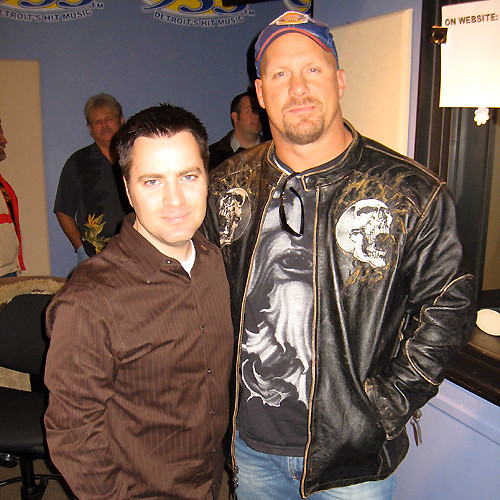In the foreground of the image, two men are posing for a photograph. The taller man on the right is wearing a blue cap with a red-lined bill and an orange or yellow logo, a gray leather jacket displaying a skull icon, and an unzipped black t-shirt with a partial skull or face design visible, specifically showing an eye. He also sports a goatee. The shorter man on the left has dark brown hair, is clean-shaven, and wears a striped brown button-up long-sleeve shirt over a white t-shirt.

In the background, there are two other men, both wearing glasses, standing against a light blue wall. To the upper right, a slide or piece of paper displays partial text reading "on website," though it is unclear which website it refers to. Additionally, part of a person in a tan and red jacket can be seen near a table. The men in the foreground are the primary focus, while the backdrop provides context about the setting being an indoor room.